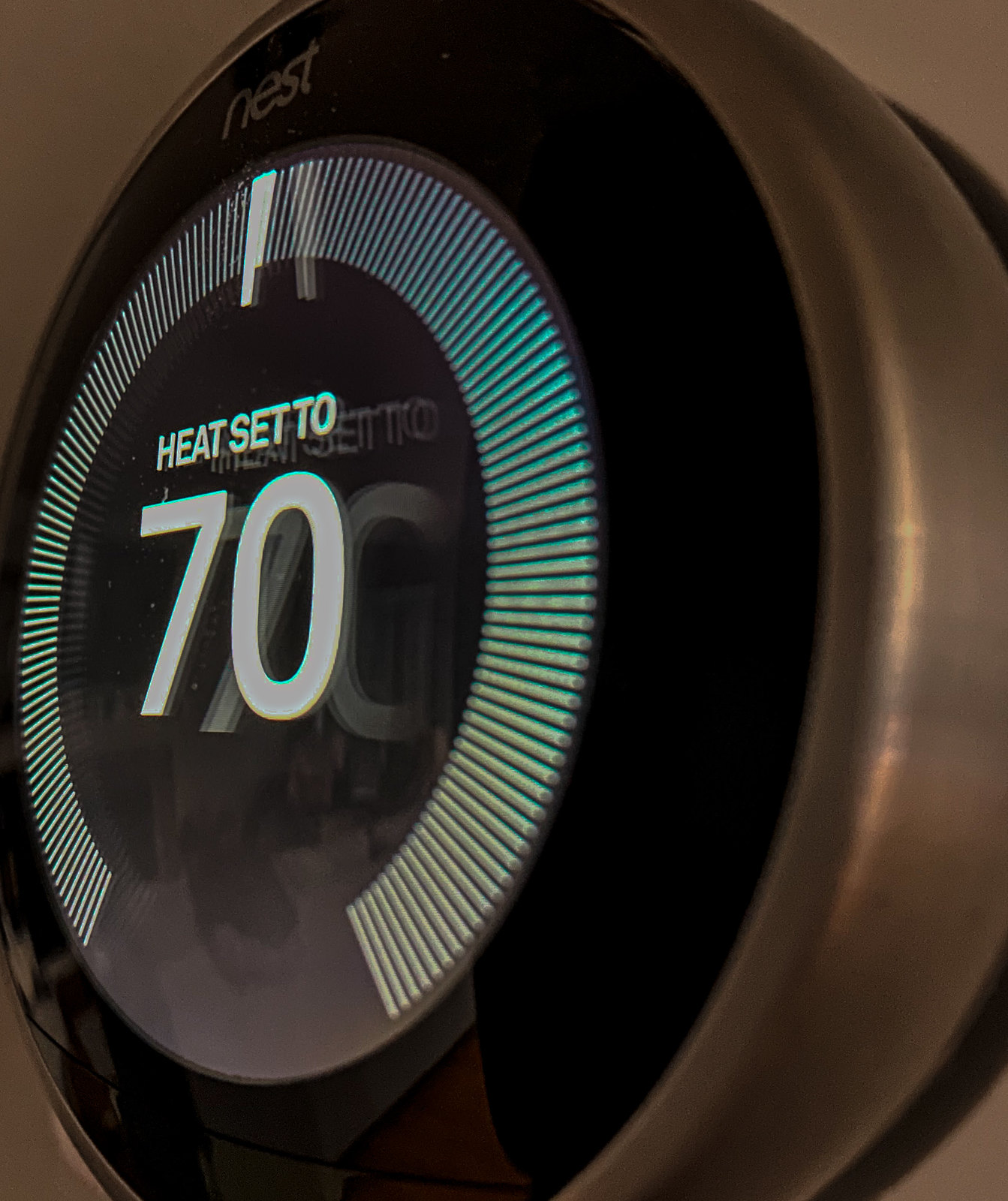This photograph captures a close-up, side view of a Nest thermostat mounted on a grayish wall. The device is slightly tilted to the left, emphasizing its sleek, modern design. The thermostat features a silver metallic outer ring that contrasts with a black display area. Prominently displayed at the top of the black section is the brand name "Nest" in a silver or white font. Below this, the display showcases a large gray circular interface. Surrounding this interface is an almost complete circle of illuminated lines, glowing in a greenish-white hue, with an opening at the bottom. In the center of the display, the thermostat reads "Heat Set To" in small font, followed by the number "70" in bold white digits. The illumination of these indicators casts a subtle reflection onto the wall behind, enhancing the visibility of the text and adding depth to the image.